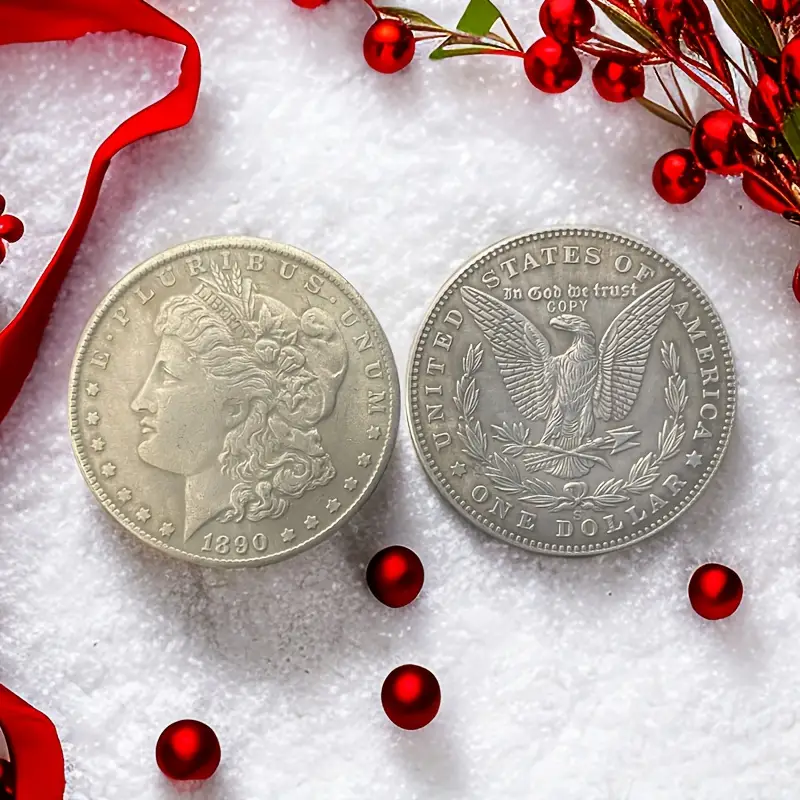This image showcases two 1890 silver dollars positioned side-by-side on a crisp white backdrop, reminiscent of snow or styrofoam. The coin on the left displays the obverse, featuring Lady Liberty facing left, adorned with a crown inscribed with "Liberty," encircled by stars. Surrounding these coins, there are scattered small red beads and metallic holly berries, enhancing the festive holiday aesthetic. A red ribbon meanders through the scene, prominently on the left and also visible intertwined with the beads in the top right corner. The reverse side of the coin on the right features a classic American eagle with wings spread, grasping arrows and an olive branch, nestled within a wreath. Both coins bear inscriptions including "E Pluribus Unum," "United States of America," "One Dollar," and "In God We Trust."